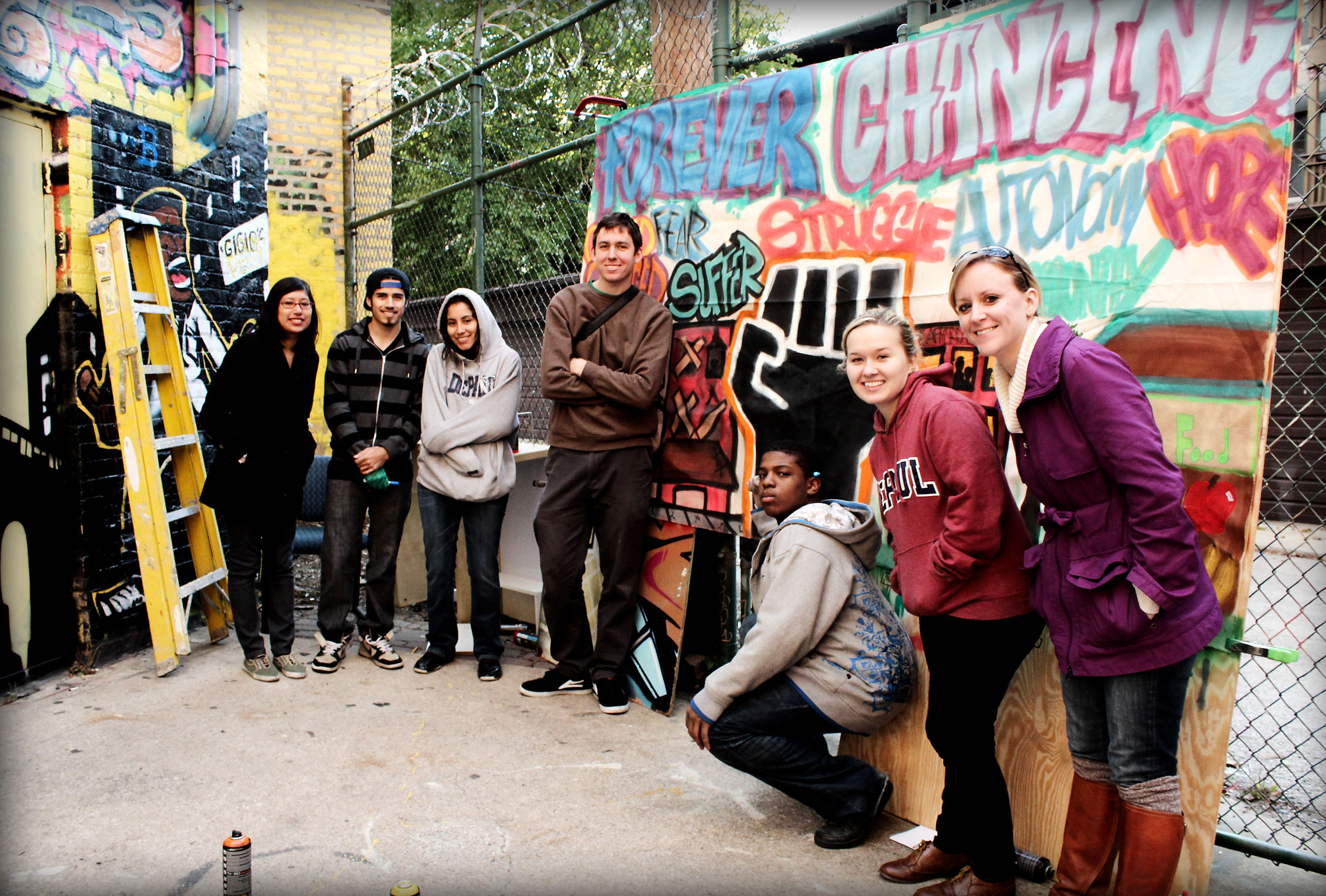In this detailed outdoor image, seven people are gathered in front of a colorful, hand-painted mural displayed on a canvas stretched over plywood. They stand by a chain-link fence topped with barbed wire. Behind the group is a yellow stone wall covered in graffiti, with a yellow ladder propped against it. The mural, which appears freshly painted with visible spray cans nearby, features the words "forever changing, fear, suffer, struggle, autonomy, hope" and a prominent black fist logo in the center. The group consists of a diverse mix: on the left, a woman in glasses, followed by a Hispanic man and woman with their arms crossed. There is a white man in brown attire, a young Black man kneeling in blue jeans and a hoodie, and two white women — one in a red sweatshirt and blue jeans, the other in a purple coat with jeans and boots. The casual and varied attire suggests they might be college students or members of a class or theater group, coming together to create or celebrate this expressive piece of art.